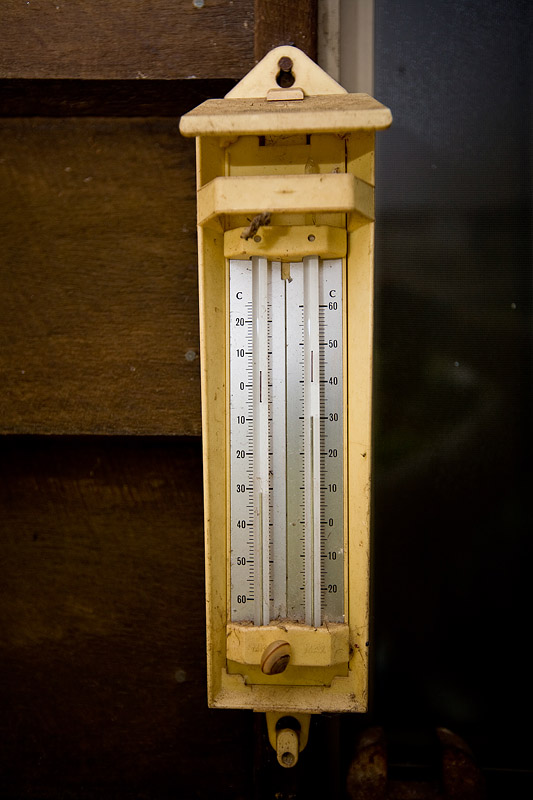Against a backdrop of weathered, dark brown wooden slats, an aged mercury thermometer takes center stage. Vertically oriented in the portrait format, the photograph captures the thermometer's off-white, weather-beaten housing, now showing signs of age and exposure. The thermometer itself consists of two mercury tubes side by side, encased within the worn exterior. Affixed to the edge of a building, the housing is secured by a single, prominent nail at its top. To the right of the thermometer is a stretch of dark, empty space, contrasting starkly with the rustic texture of the slats on the left, emphasizing the solitary, utilitarian beauty of the old weather instrument.